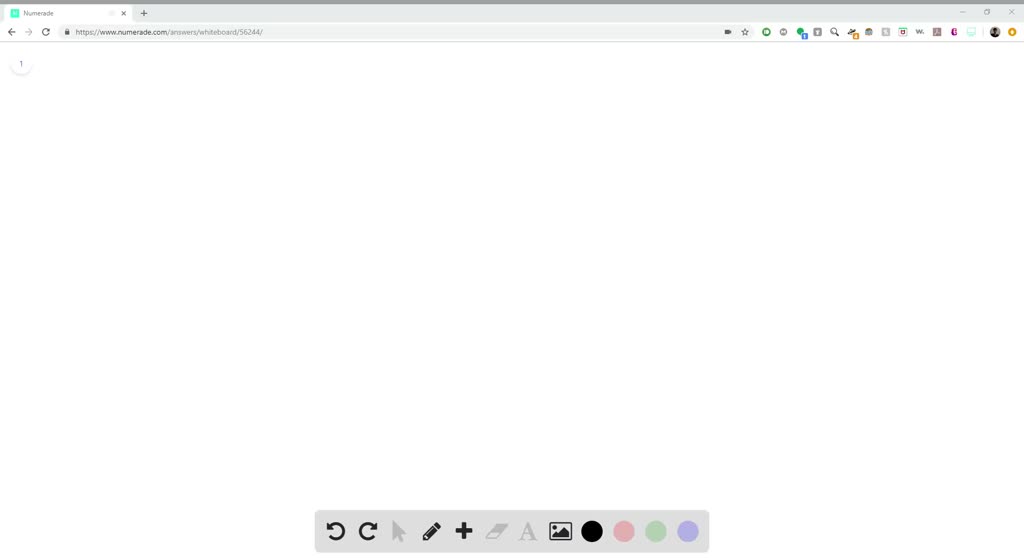The image is a screenshot of a website, prominently featuring the top portion of a web browser window. The majority of the screenshot highlights the browser's user interface elements. At the very top, there's a dark gray line extending across the width of the image. Below this, the lighter gray standard browser bar is visible.

On the upper left of the bar, a white tab is opened. The tab displays a small green square icon next to a tiny, black text that appears to read "Numerate." To the right of this, there's a gray "X" to close the tab. Adjacent to the tab is a black arrow on the gray background, followed by a black plus sign for opening new tabs.

On the far upper right corner of the browser, standard window buttons are present: a minimize icon, a reload icon, and a close window "X" icon.

The URL bar is centrally positioned and starts on the left with a black back arrow, a gray forward arrow, a reload button, and a black padlock icon. The URL displayed is "numerate.com." 

To the far right of the URL bar, there is a series of icons: 
- A video camera icon
- A star icon
- A green icon
- A gray icon
- A green icon containing a blue square with the number "1" in it
- Another gray icon
- A search icon resembling a magnifying glass
- A gray icon with an orange square displaying a white digit that is too blurry to read
- A gray outline square that seems to resemble the McAfee logo
- The WordPress logo
- The Adobe logo
- An icon with red coloring
- An icon with blue coloring
- A user profile icon
- An orange icon

At the very bottom of the image, there's an editing or formatting toolbar. It features:
- A black reload button on the left
- Another black reload button on the right for navigating back and forward
- A diagonal gray arrow
- A black pencil icon
- A black plus sign
- A gray eraser
- A gray letter "A"
- A black image icon
- Four colored dots (black, pink, green, and purple)

This detailed layout captures the essential elements of the screenshot, emphasizing the various icons and interface components visible in the browser and toolbar.